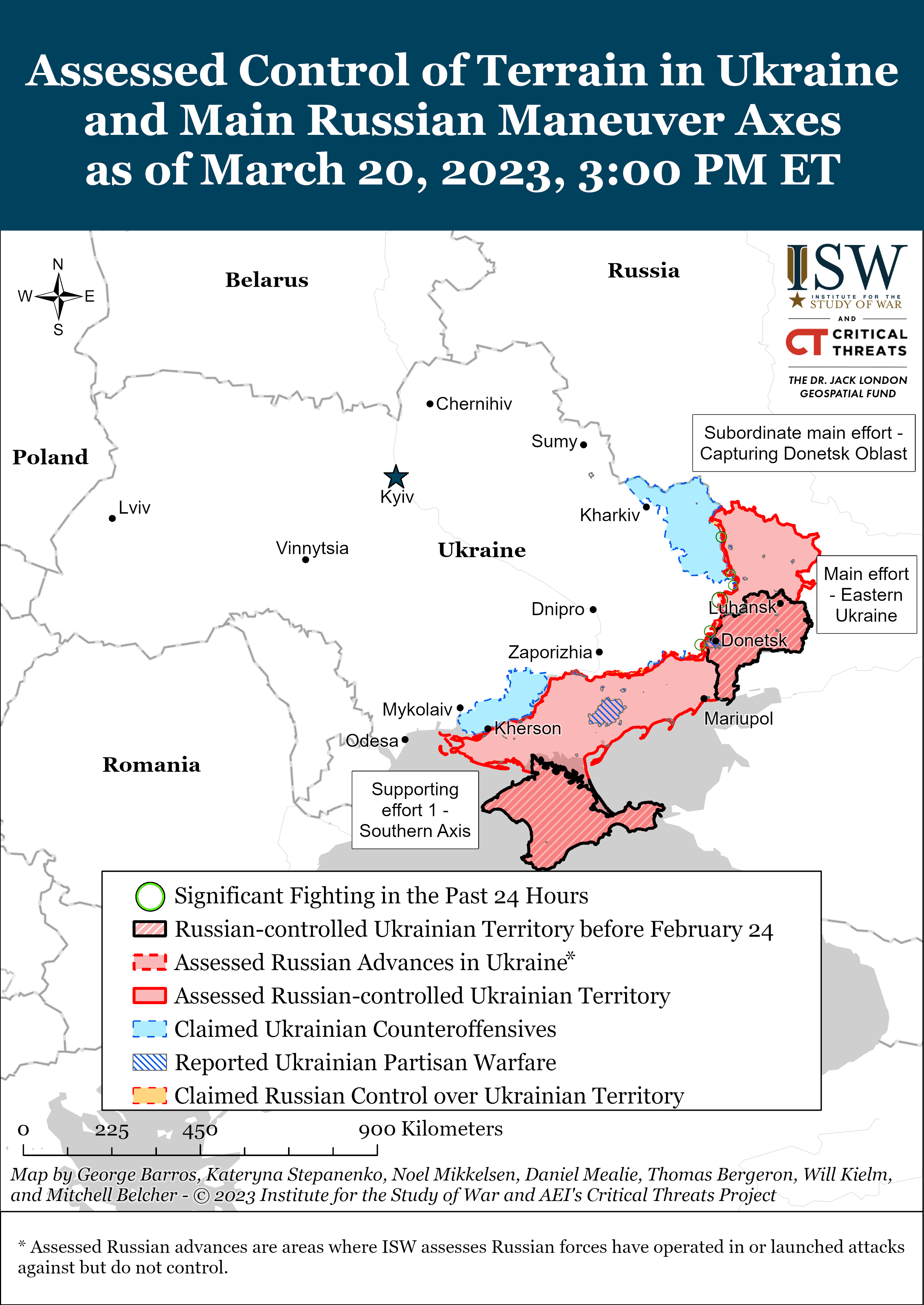The image is a detailed map titled "Assessed Control of Terrain in Ukraine and Main Russian Maneuver Axes as of March 20th, 2023, 3 p.m. ET," prominently displayed in white text against a dark blue background. The map encompasses regions including Ukraine, Russia, Belarus, Poland, and Romania, with specific focus on Ukrainian cities.

The map uses a variety of colors and patterns, explained in a legend below the map, to highlight different control zones and military activities:
- Solid red areas indicate Russian-controlled territories as of February 24th.
- Red striped areas represent assessed Russian-controlled Ukrainian territories.
- Blue areas denote claimed Ukrainian counter-offensives.
- Purple areas mark reported Ukrainian partisan warfare.
- Yellow-orange, though listed in the legend for claimed Russian control, does not appear on the map.

The northern, eastern, and southern regions of Ukraine show significant use of red and red-striped patterns, indicating substantial Russian influence and activities in these zones. The map also includes markers and text detailing subordinate main efforts, such as capturing Donetsk Oblast and main efforts in eastern Ukraine, along with supporting efforts in the southern axis.

Additionally, the map credits various sponsors and includes a legend with symbols in green, red, blue, and yellow-orange, aiding in the interpretation of control dynamics as per the latest assessment date.